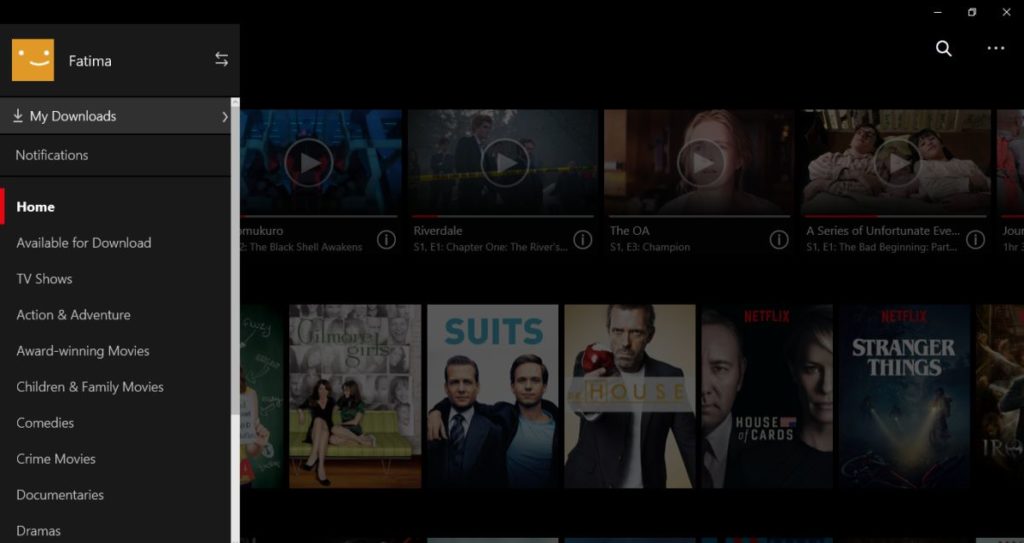The left side of the image features an orange square with a smiling face, labeled as "Fatima." Adjacent to it, there is a rectangle representing "Grace" and another labeled "Mandela," followed by "Identifications."

The user interface displays various categories, including:
- Home
- Available for Download
- TV Shows
- Action & Adventure
- Award-Winning Movies
- Children & Family Movies
- Comedies
- Horror Movies
- Documentaries
- Dramas

Prominent images include:
- Mecca
- Southern Riverdale
- The O.A.
- A Series of Unfortunate Events

For "Riverdale," the display specifies:
- Season 1, Episode 1: Chapter 1
- Season 1, Episode 3

Other highlighted shows and images:
- "Gilmore Girls," featuring a memorable scene
- An individual seated on a couch, suggested to be from the same show
- "Suits," displaying two people in suits, along with separate images showing one person wearing a suit and another person holding an armband
- "House," featuring Dr. House
- "House of Cards," showcasing two main characters
- "Stranger Things," with an associated image
- An ambiguous image possibly depicting "Iroh," potentially from "The Legend of Korra"

Overall, the interface provides a detailed and diverse array of television shows and movies available for viewing.